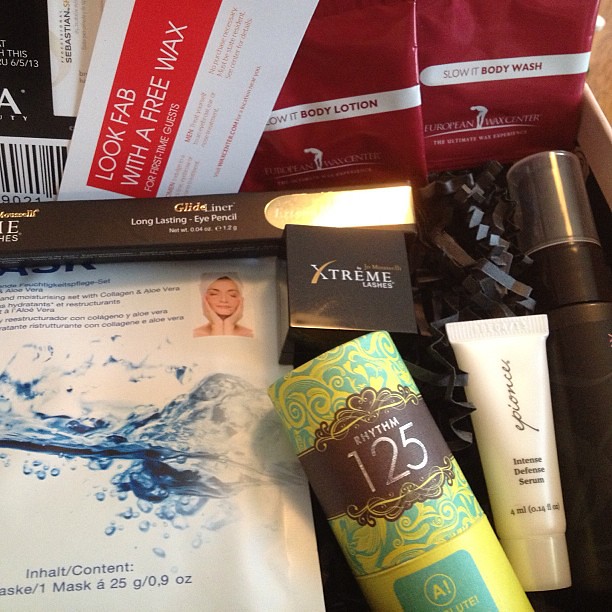The image depicts a cluttered assortment of beauty products, likely contained within a gift or sample box. In the left-hand corner, there's a card with a white background, offering a "Look fab with a free wax" promotion for first-time guests. To the right of the card is another card with a red background and white text advertising "Body lotion." The box includes various items such as a clear, tan bottle labeled "Defense Serum," a brown bottle, a long-lasting eyeliner pencil by the brand Glide, and a box of Extreme Lashes. Additionally, there are tubes and packages of face cream, hydrating masks, a body wash, and other cosmetic samples. The products are nestled atop confetti-like material, adding to the presentation's festive, gift-like appearance.